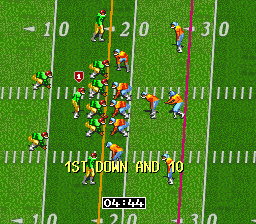This screenshot captures a crucial moment in a football video game where the play is about to commence. The red and green teams are lined up at the line of scrimmage, which is positioned approximately at the 18-yard line. It is first down with 10 yards to go, and the game clock shows 4 minutes and 44 seconds left in the quarter. The quarterback is in position, poised to call for the snap, while the wide receivers are spread out across the field, ready to execute the play. The offense is geared up to make a push towards the opposing end zone.